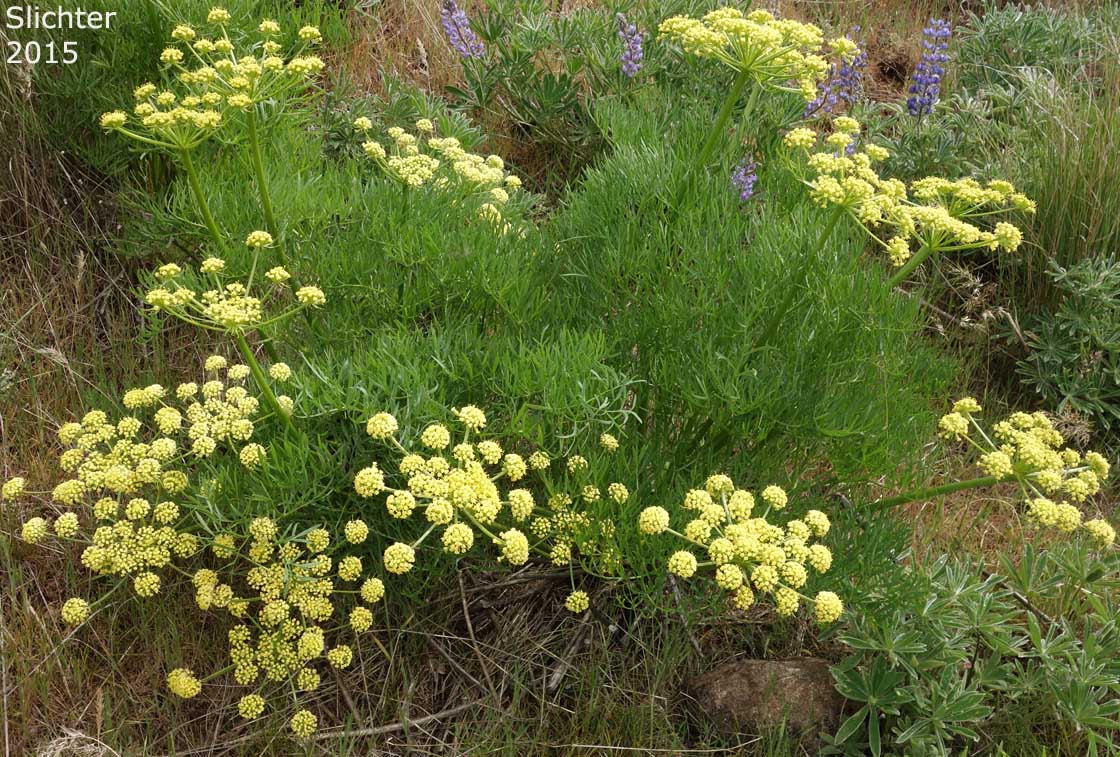This aerial photograph captures a wild hillside adorned with clusters of vibrant yellow and purple flowers. The perimeter of the image shows a lot of gray, decaying grass and twigs, while the center reveals a lush cluster of greenery. Emerging from this greenery are numerous thin-stemmed, starburst-design clusters of yellow flowers, numbering about nine or ten. Interspersed among the yellow blooms are several tall, cone-shaped purple flowers that stand out vividly against the surrounding grass. In the foreground, a large rock is partially obscured by the foliage. The upper left corner of the image displays the text "Slichter 2015" in white lettering, possibly indicating the date or author of the photograph.